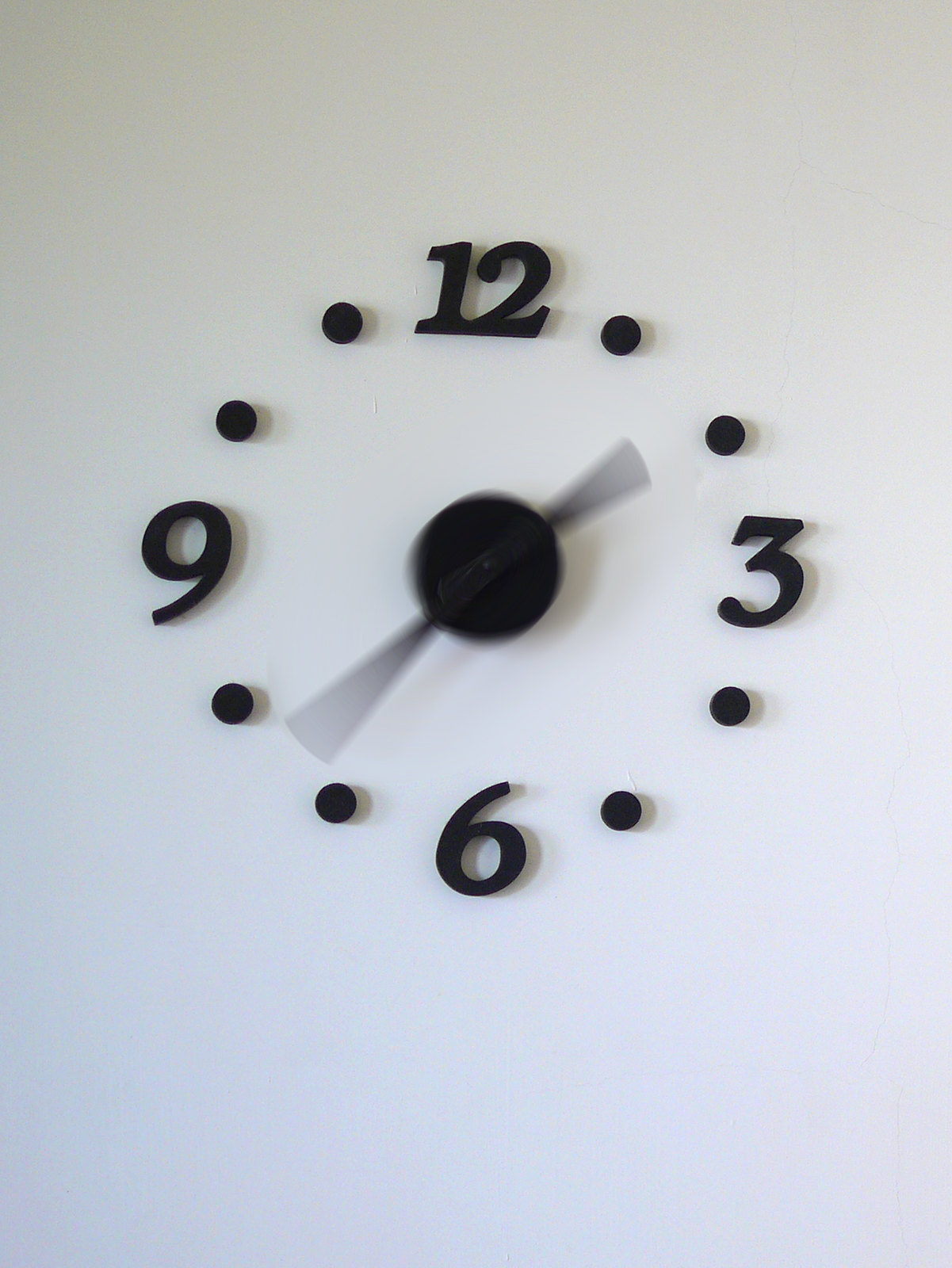This image depicts a clock, likely a wall clock based on its design. The photograph, or possibly a high-quality product rendering, shows a close-up of the clock's face with no visible edges or borders. The clock features a minimalist design with a black casing and a face that appears to be gray or off-white. The dial includes numerals at the 12, 3, 6, and 9 positions, while the remaining hours are marked by small dots. The clock is stripped of a second hand, possessing only slender minute and hour hands that extend from a prominent circular hub at the center. The clean and simple aesthetic highlights the clock's functional elegance.